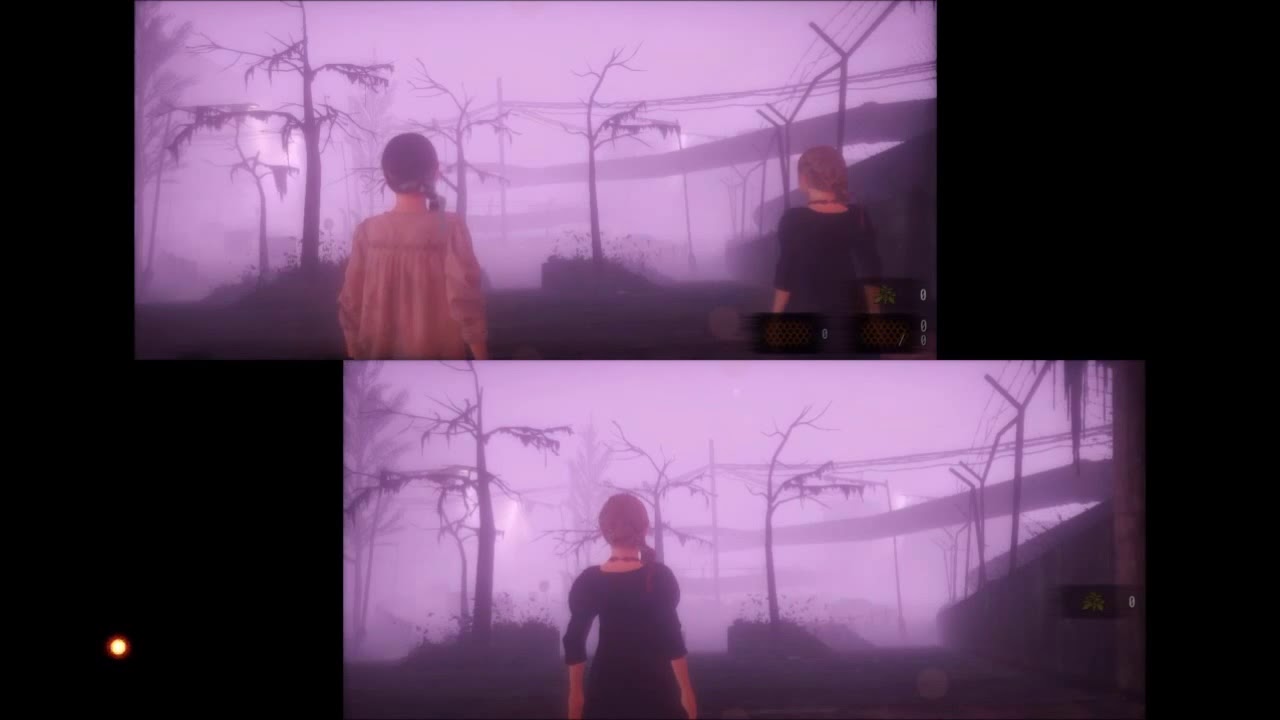In this horizontally rectangular image set against a solid black background, there are two distinct screenshots stacked vertically, depicting a foggy, apocalyptic scene with muted colors leaning towards gray and purple. Both images feature a hauntingly misty landscape with dead trees and large pipes, enhancing the eerie atmosphere. In the top screenshot, two female characters stand prominently. The girl on the left wears an orange, light dress with sleeves extending past her elbows and her hair pulled back in a ponytail. The girl on the right has red hair, wears a black dress with a necklace, and her sleeves are also long. She too has her hair pulled back in a ponytail. The bottom screenshot is a cropped version of the top, focusing solely on the girl in the black dress, who appears against the same desolate background. Both images include game interface icons and numbers, indicating they are likely clips from a video game.